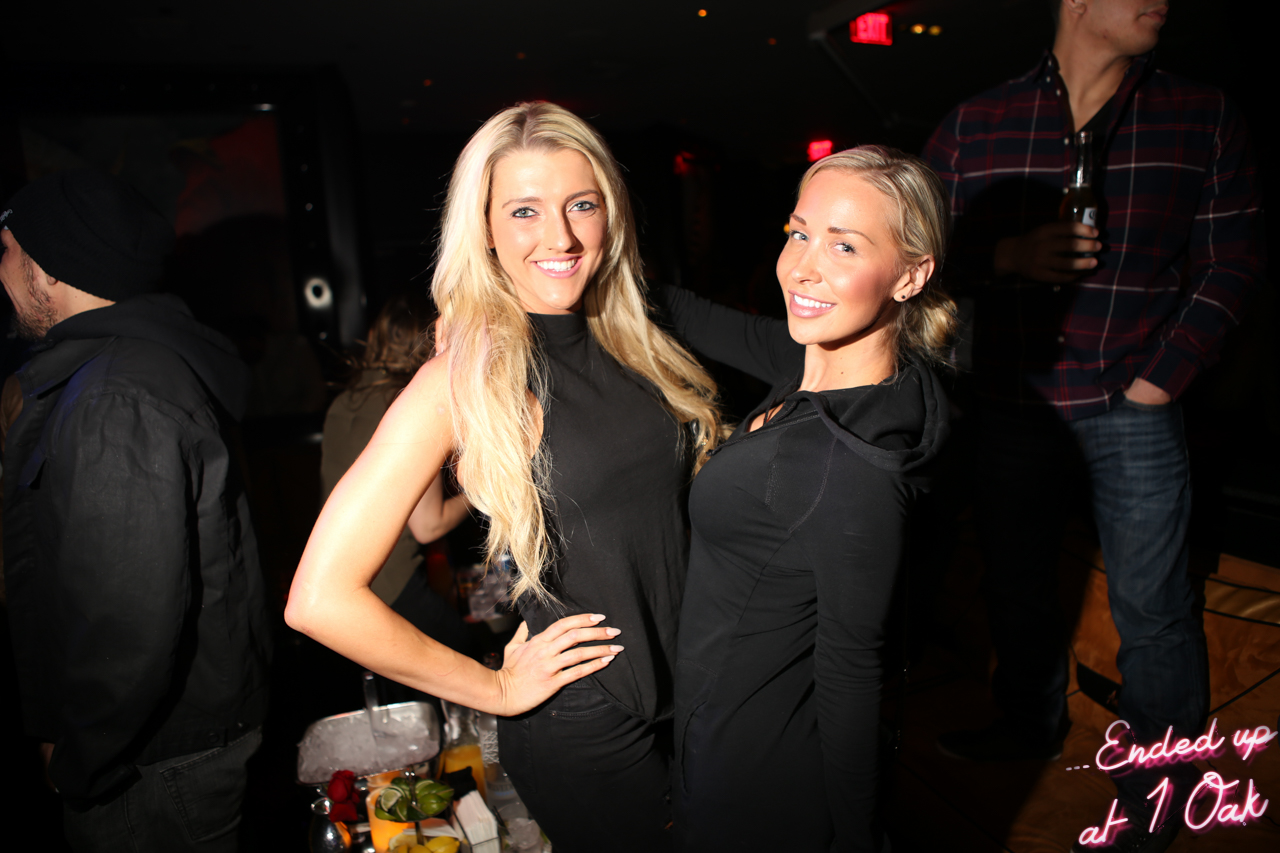The photograph captures a lively, nighttime scene at a dance club or bar, possibly "One Oak," as indicated by the cursive inscription in hot pink and white script text in the lower right-hand corner. The focus is on two women in the foreground, both wearing black attire. The woman on the left sports long, flowing blonde hair, a sleeveless, high-collar black shirt, and black pants, with one hand placed confidently on her hip. To her right, another woman, also with blonde hair styled in a bun, has her arm draped around her companion's shoulder and wears a black, zippered-up hoodie. Both women are looking at the camera and smiling. In the background, to the right, a man in a blue and red plaid shirt and jeans holds a beer bottle, partially obscured with one hand in his pocket. To the left, another individual in a black hat and jacket looks away from the camera. The dim, ambient lighting and background activity suggest a bustling party or dance atmosphere.